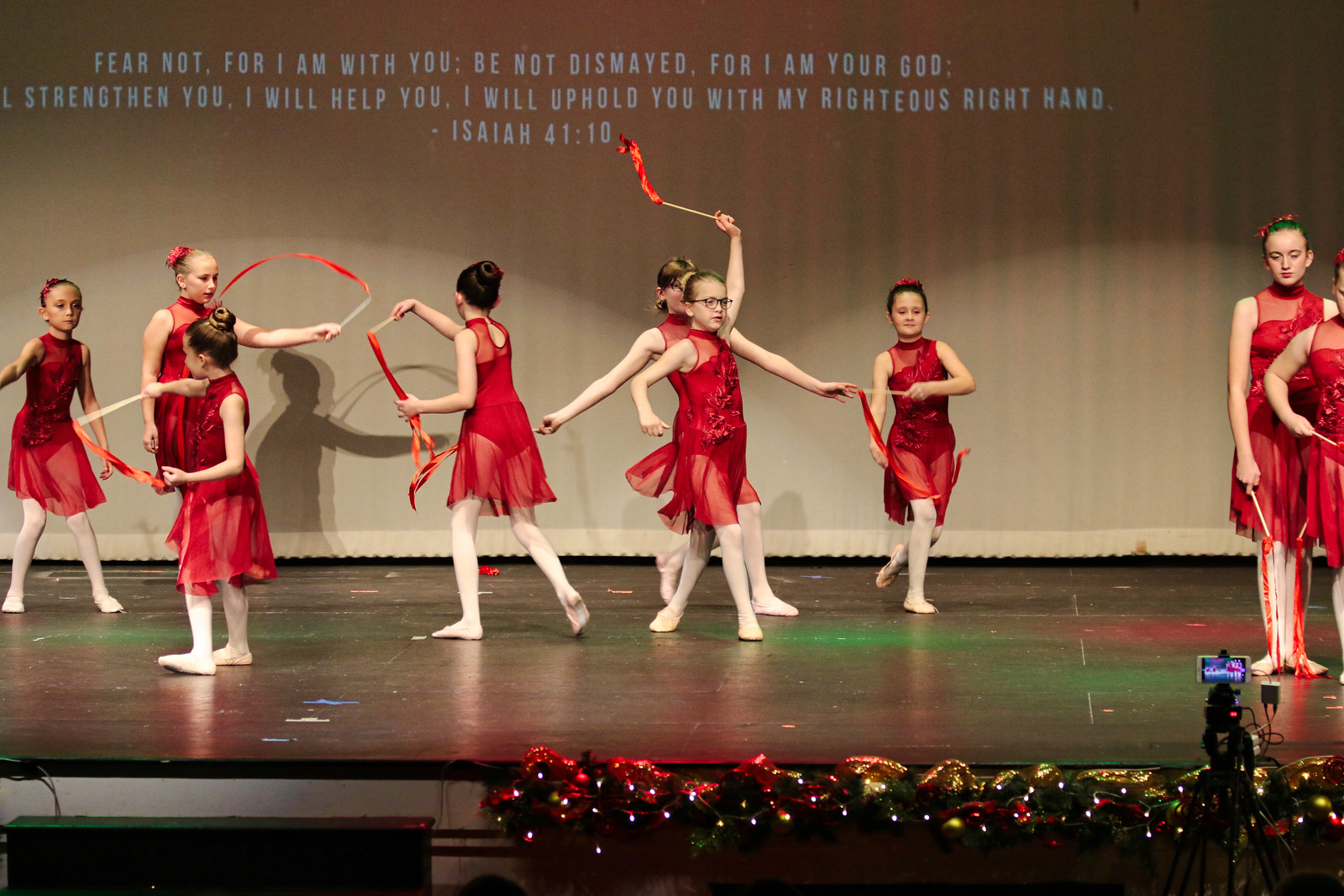The image depicts a group of nine young girls on a wooden stage, performing a dance. Each girl is dressed identically in a vibrant red dress with sheer, gauzy skirts that reach up to their necks and are sleeveless. The dresses feature appliques of red flowers that run diagonally from the shoulder to the waist. Complementing their attire, the girls wear light pink tights and pink ballet shoes. Some hold ribbon wands with red ribbons tied at the end, which they twirl gracefully during the performance. Their brown hair is neatly tied back. 

The stage appears elaborately decorated for Christmas, with colorful lights and festive decorations adorning the front. A tripod camcorder is set up, presumably to record the performance. Green lights illuminate parts of the stage, enhancing the festive atmosphere. In the background, a dark backdrop with a projected white text reads: "Fear not, for I am with you; be not dismayed, for I am your God. I will strengthen you, I will help you, I will uphold you with my righteous right hand. - Isaiah 41:10". The text provides an inspirational touch to the scene, underscoring the theme of support and courage.